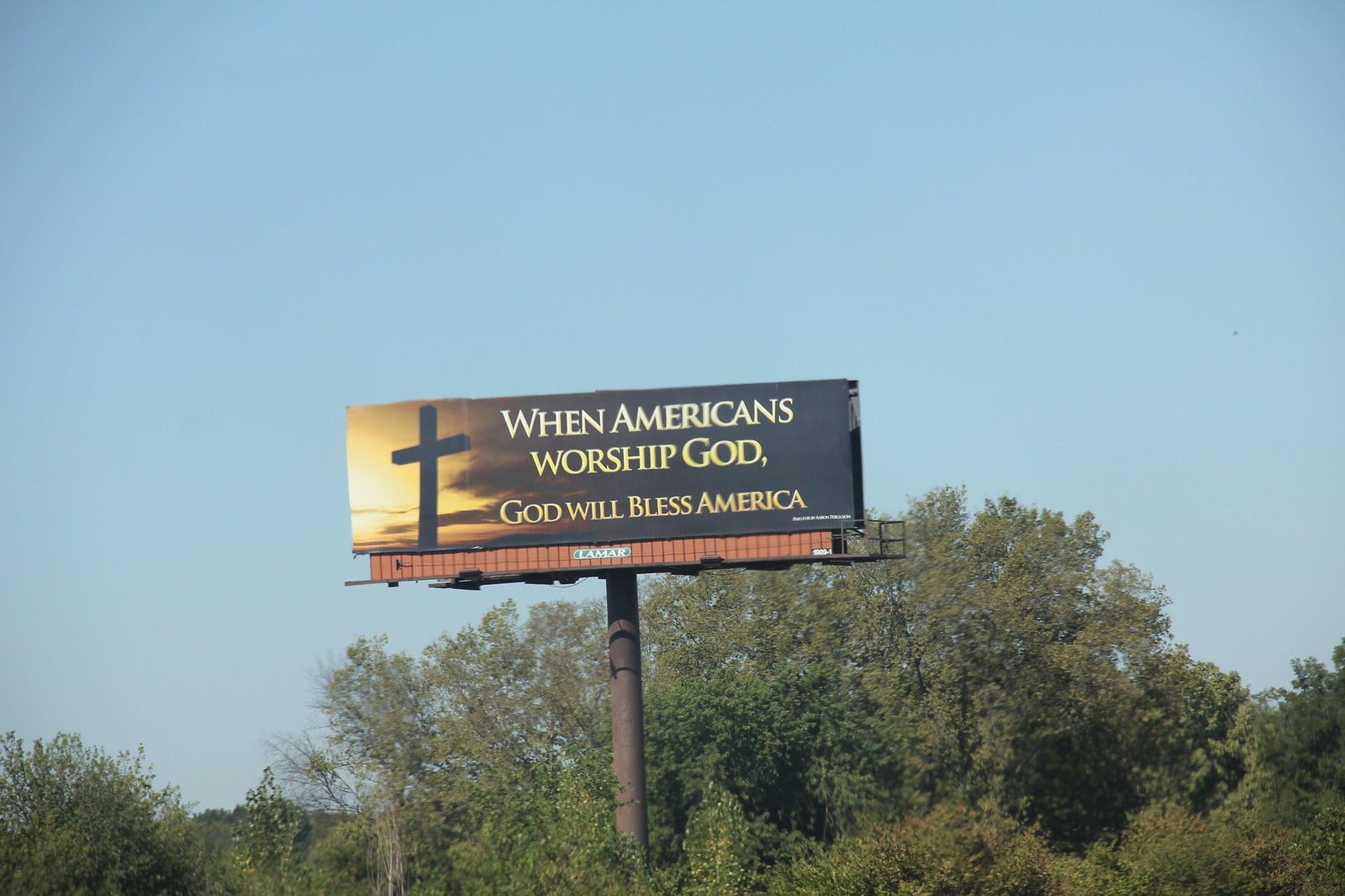This is a color photograph of a billboard captured from an upward angle, prominently centered in the image. The billboard stands on a round brownish-red pole, and the base of the structure features an orange hue with "Lamar" written in white text on a green oval. The billboard itself is horizontally rectangular and reads in gold writing, "When Americans worship God, God will bless America." The background of the billboard ranges from a golden sunset on the left, featuring a large, dark brown cross silhouetted against the bright light. This transitions to a dark, cloudy sky dominating the right side of the billboard. Below the billboard, a line of trees stretches from left to right, none of which rise above the midpoint of the structure. The overall backdrop beyond this scene includes patches of clear blue sky.